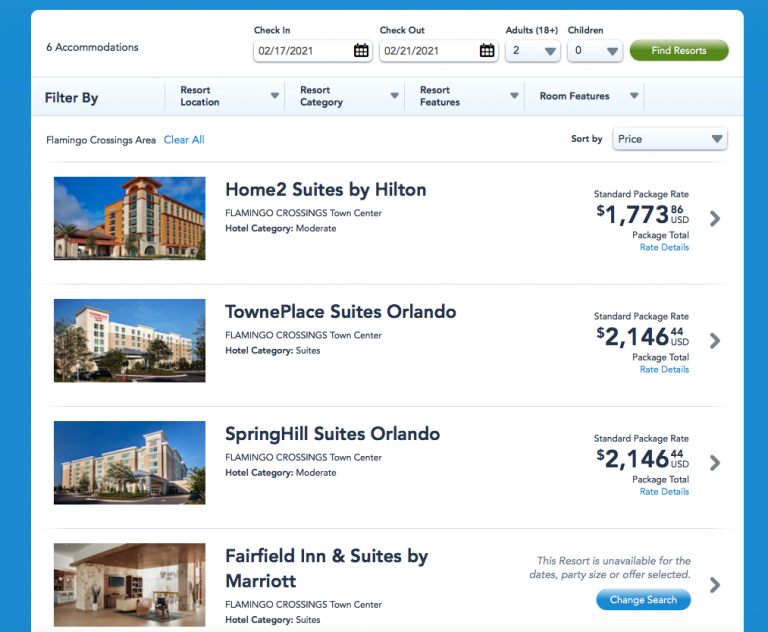The image depicts a travel website interface similar to Priceline or Orbitz, viewed on a desktop. The page highlights booking details and choices available for a resort stay. Specifically, the check-in price is set at $217.20, and the check-out price at $221.20 for two adults. A prominent green "Find Resorts" button is visible, and the top of the page features menus and filter options. Users can filter their search by resort location, resort category, resort features, and room features.

Below the filters, four listings are displayed, each accompanied by a thumbnail image of the location and the property's building. The listings and prices are as follows:
1. **Home 2 Suites by Hilton**: Priced at $1,773, labeled as the package total for the standard package rate.
2. **TownePlace Suites, Orlando**: Priced at $2,146, labeled as the standard package rate.
3. **SpringHill Suites, Orlando**: Also priced at $2,146, labeled as the standard package rate.
4. **Fairfield Inn & Suites by Marriott**: Indicated as unavailable for the selected dates, party size, or offer, with an option to change the search.

The listings are presented in a scrollable menu format, with only four visible entries in the current view.